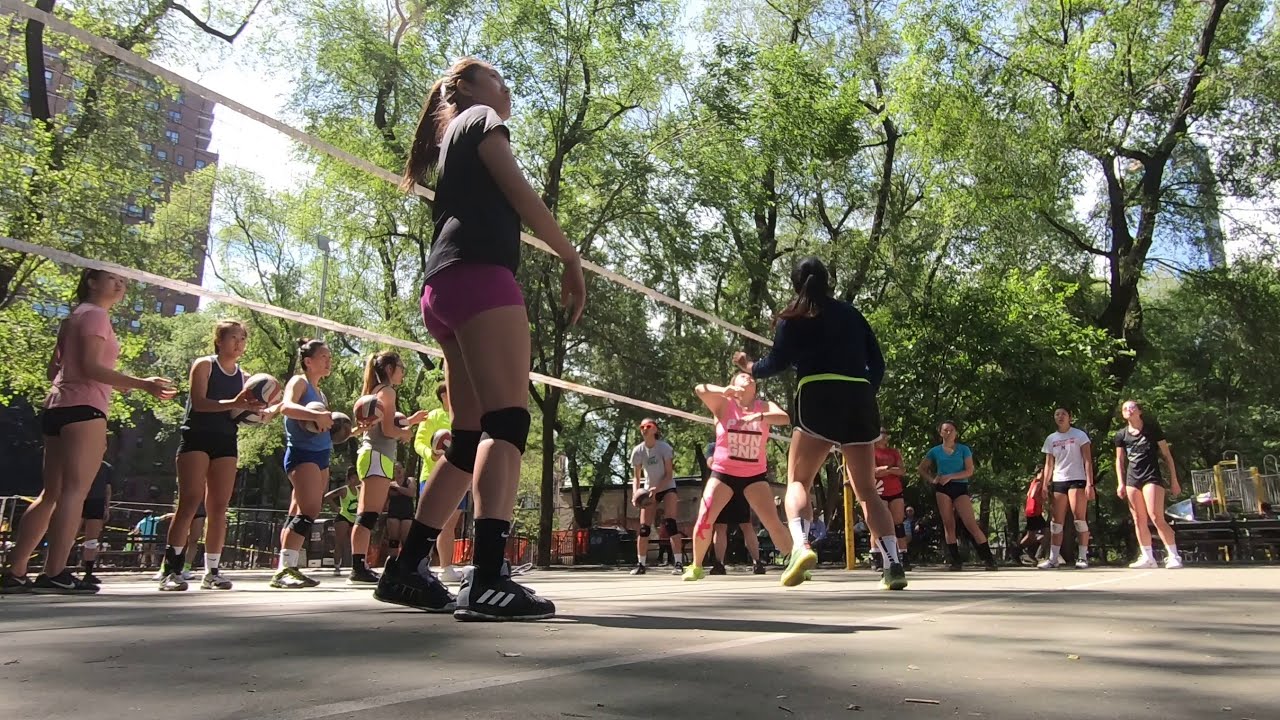The image showcases an outdoor volleyball practice session, taken from a low angle as if the camera were placed on the ground looking up. The scene is set on a concrete court in a lush urban park, surrounded by early-blooming trees and tall city buildings, hinting at a large metropolitan area like New York City. 

A multitude of teenage girls, well over a dozen, are engaged in various stages of play and preparation. Dominating the scene is a white volleyball net, highlighted with white straps on top and bottom, stretching horizontally across the image. The netting itself appears to be black. 

In the foreground, a player in a pink t-shirt and black shorts stands out, while another player with a ponytail, dressed in a black long-sleeved shirt, black shorts with a white stripe, gray tennis shoes, and white socks, appears ready to react to an impending volley. Also prominent is a woman with a gray shirt, red slacks, black socks, and distinctive black shoes with three white stripes, accentuated by two black knee bands. 

To the right of her, a line of focused girls in varied outfits—black shorts, turquoise top, red top, gray top, and a combination of light green shorts and tops—extends across a third of the picture. On the opposite side of the net, another player holds a volleyball, poised for action. 

The sky above is a picturesque blue with scattered white clouds, complementing the vibrant atmosphere. Beyond the court, signs, a potential road, distant figures, and additional park structures add to the urban park setting, with another volleyball net visible on the left, indicating multiple courts in use.